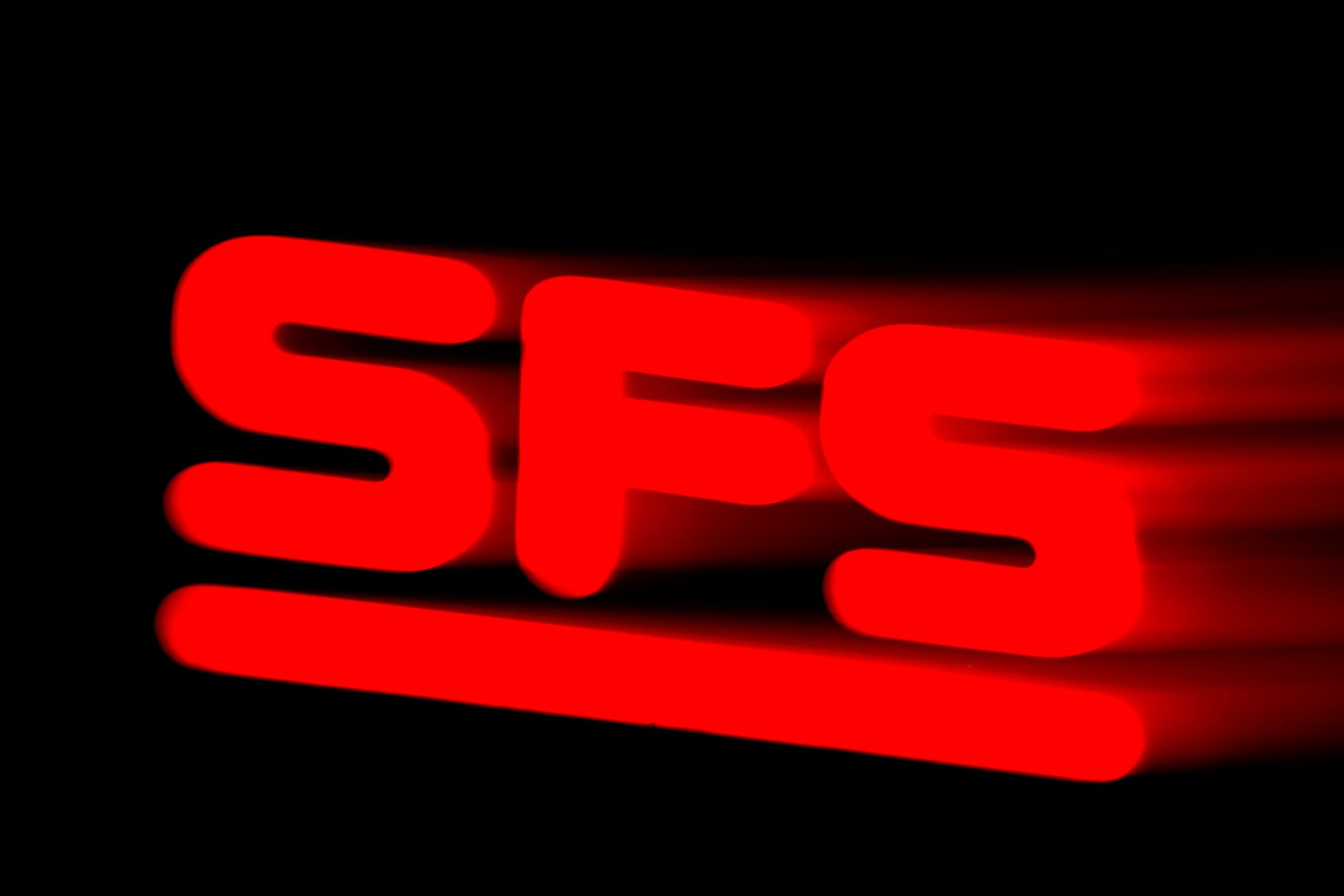The image displays a brand logo set against a solid black background, positioned centrally. The focal point of the design is the letters "S.F.S." rendered in a bold, red, science fiction-like font. These letters are underlined by a thick red bar with rounded ends. An artistic motion effect is present, as the letters and the underlining bar create a trail of red blur behind them, giving the impression of speed and movement from right to left. The dynamic design, solely featuring black and red colors, evokes a neon effect, making it striking and memorable. This logo, due to its centralized and detailed nature, is likely designed for a company, suitable for use on business cards or websites.